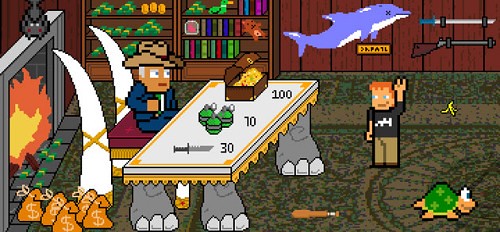This image is a screen capture from a classic early 80s video game, featuring simplistic, pixelated graphics typical of Atari games from that era. The scene is set in what appears to be a hunter's den or shop with brown wooden walls adorned with green, black, and grayish trim. Centered in the foreground is a white, rectangular table with gold trim and supported by the lower legs of an elephant. On the table lie three items: a knife, three green grenades, and a small chest filled with gold coins, each marked with the numbers 30, 10, and 100 respectively.

To the left of the table stands a man in a blue suit and cowboy hat, sitting on a bench with a red cushion trimmed in gold. Elephant tusks flank either side of his seat. Directly across from him, to the right of the table, is a boy with orange hair wearing a black shirt, tan pants, black shoes, and raising his left arm, possibly in greeting or signaling.

In the background to the left, a large gray fireplace with a red and yellow flame crackles, with money stacked in front of it. Above the fireplace is a bookcase. To the right, the walls display a purple dolphin facing right with a white belly and a weapon rack holding a long knife with a blue handle and a gun with a brown frame and silver barrel. Amid these decorations, a digitized turtle moves rightward in the bottom right corner next to a grouping of four brown money bags tied with yellow string, all marked with a money symbol. Bonanza elements like an additional bat on the floor enhance the rich atmosphere of this pixelated hunter's den.